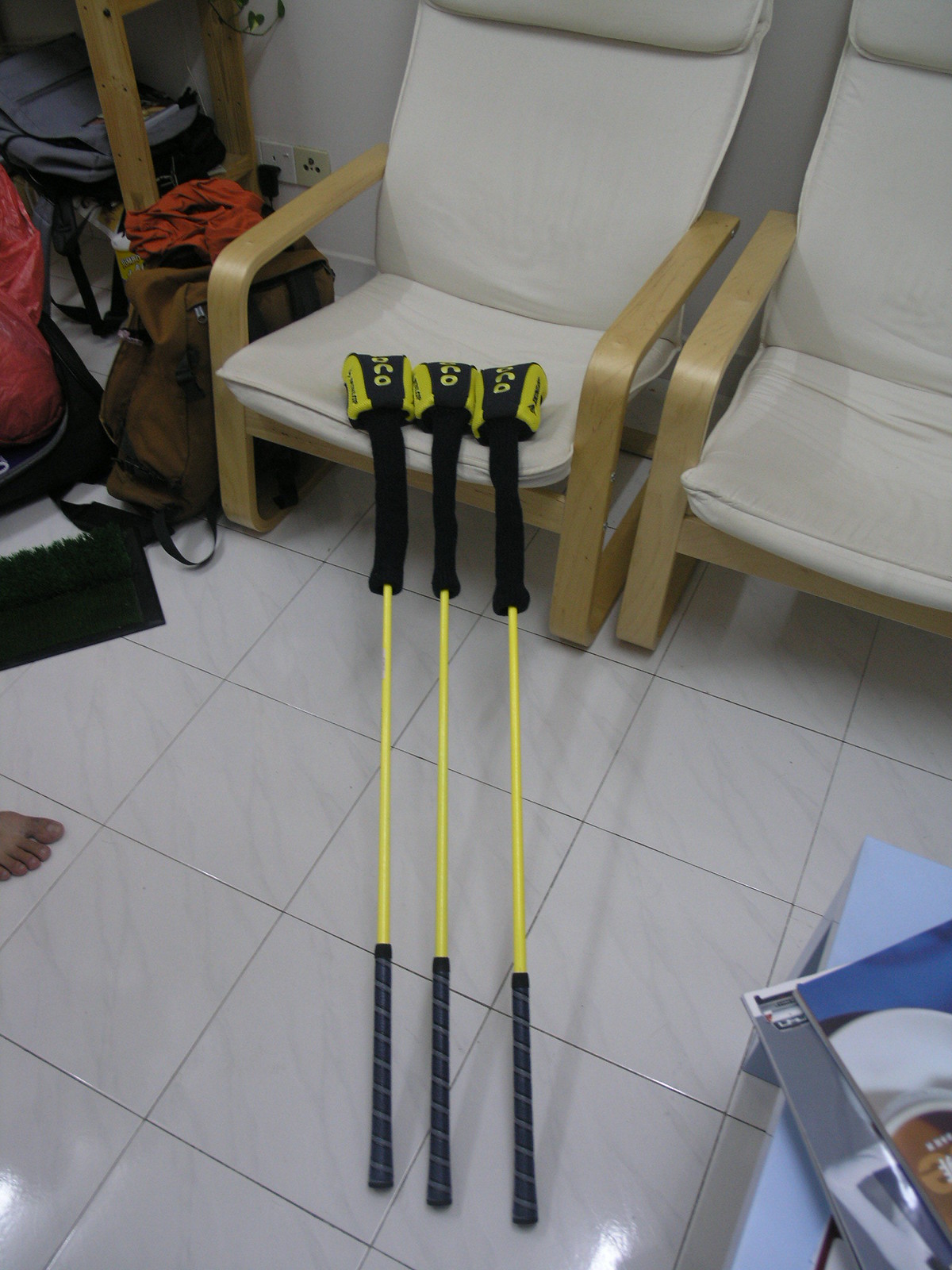In this detailed indoor photograph, three golf clubs are prominently featured, leaning against the leftmost of two off-white linen chairs with simple wooden frames and armrests. The scene is set against a grey back wall, with clean white tile flooring interspersed with black grouting. The golf clubs, thin and yellow with black fabric "socks" covering their heads, rest on the seat cushion, angling down to the floor where their rubber grips touch the tiles. 

To the left of the image, near the edge, the bare toes of an unseen person peek into the frame. Above this, a brown backpack slightly ajar reveals a red fabric inside, while a shelf nearby holds additional bags, including a red one with black handles and a gray one. To the right, a blue table stands with a few magazines on top. The setting, which suggests a cozy, possibly domestic environment, is punctuated by various details like electrical outlets with cords plugged in, reinforcing the lived-in feel of the space.